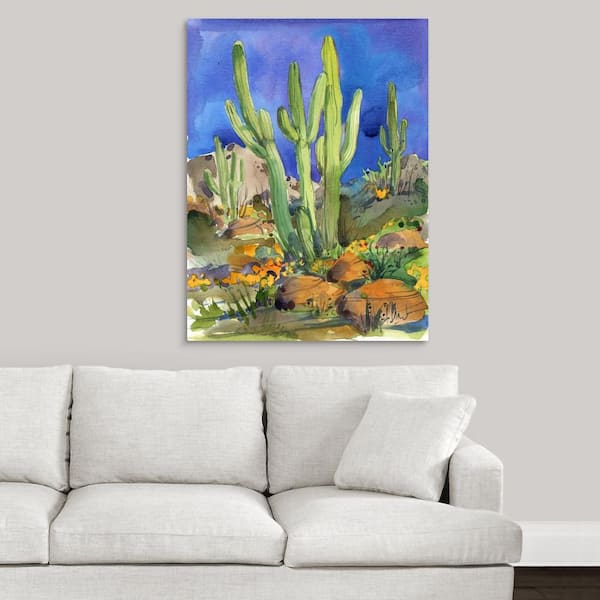This is a photo showcasing a stylish living room with detailed decor. The room features a light gray wall with a white baseboard trim, complementing the brown hardwood floors. A white three-seater couch, complete with matching white cushions and a square pillow, is placed against the wall, creating a soothing and plain visual foundation. Hanging above the couch is a striking rectangular painting of a vibrant desert scene. The artwork vividly depicts three tall cacti with green stems against a backdrop of a dark blue sky, indicating late in the day. The foreground teems with desert flowers in shades of yellow, orange, and brown mounds of sand, adding bursts of color that make the room pop. The painting's vibrant colors juxtaposed with the muted tones of the couch and wall, elevate the aesthetic of the room, making it visually appealing and lively.